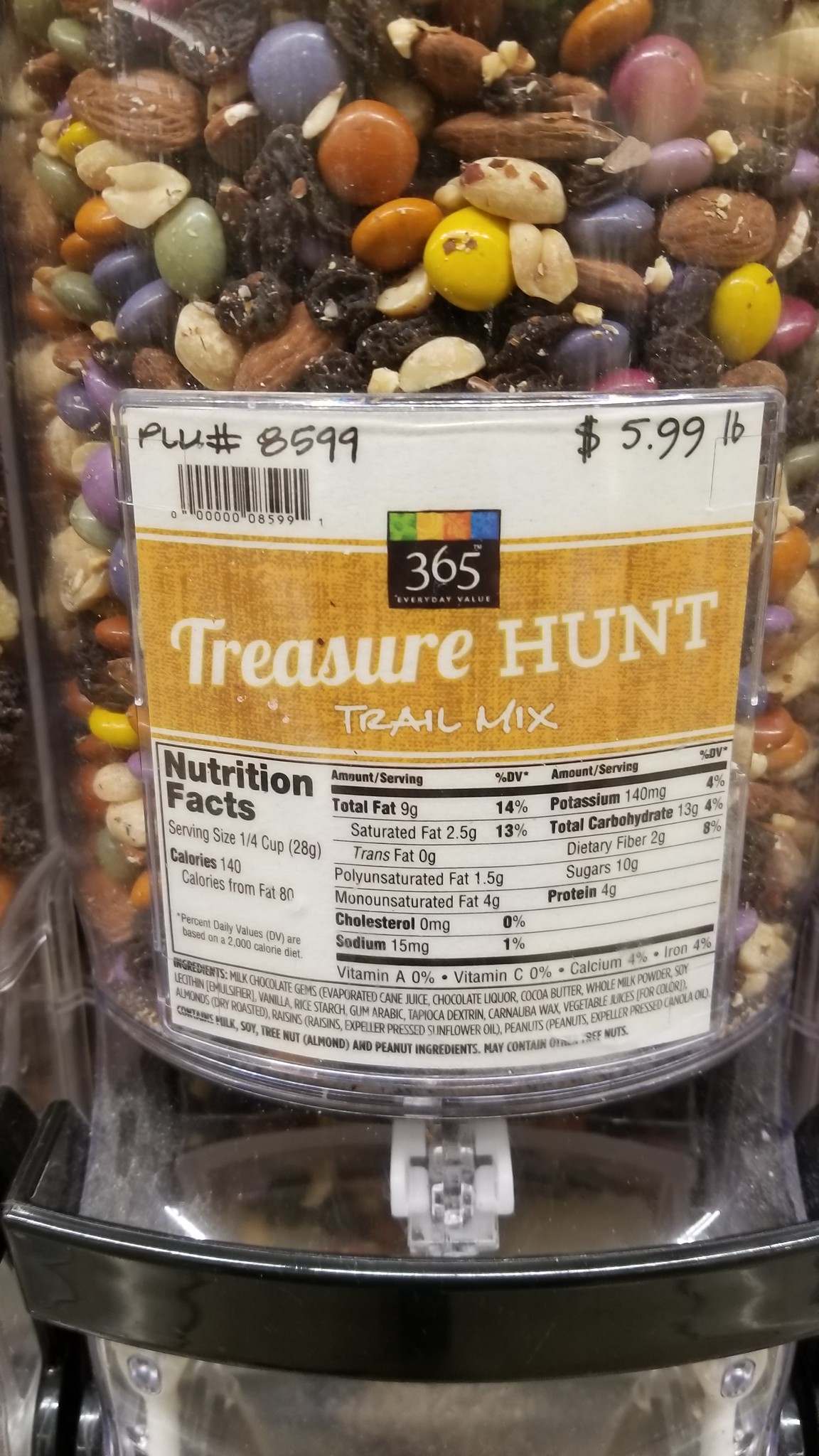This close-up image captures a front-facing view of a candy dispenser. The main container, which is prominently featured, is filled with a trail mix that includes chocolate M&M pieces, peanuts, and raisins. A notable tag is attached to the front of the dispenser. The tag, written in ink, displays the price "$5.99 per pound." Additionally, a brown banner across the tag reads "Treasure Hunt Trail Mix," accompanied by the nutritional facts of the mix. Below this tag is the dispensing mechanism, featuring a metal bar that likely facilitates the release of the trail mix into a container for purchase.